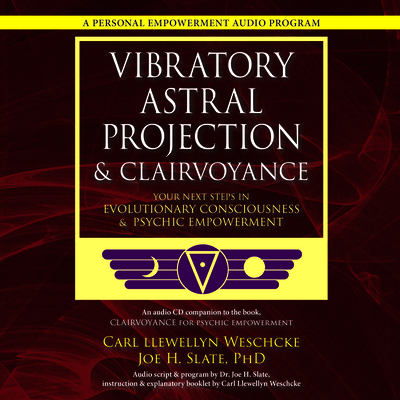The image depicts the cover of a vibrant personal empowerment audio program. Dominated by a dark brownish-purple background with wine-red swirls reminiscent of flowing satin, the cover reads "A Personal Empowerment Audio Program." The prominent main heading, "Vibratory Astral Projection and Clairvoyance," is accompanied by a subheading, "Your Next Steps in Evolutionary Consciousness and Psychic Empowerment." The authors, Carl Llewellyn Weschke and Joe H. Slate, PhD, are credited below. Accentuated by yellow horizontal stripes, there is an eye-catching logo featuring a triangle with a small sphere inside, flanked by a crescent moon on the left and a full sun on the right. The fonts stand out in white and yellow, making the text easily legible.